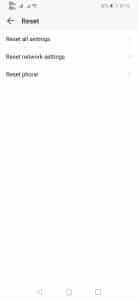A blurry screenshot depicting a phone settings page with three distinct rows of options. Each row likely corresponds to different reset settings, though the text is largely illegible due to the image quality. The first option appears to read "Reset All Settings," followed by "Reset Network Settings" for the second, with the third seemingly labeled "Reset Phone." These options suggest the user is navigating through their phone to possibly reset either specific configurations—such as network settings—or return the device's settings to their default state. Visible at the top corners of the screen are typical phone status icons, including a barely discernible battery indicator on the top right, reinforcing that this is indeed a mobile device interface.